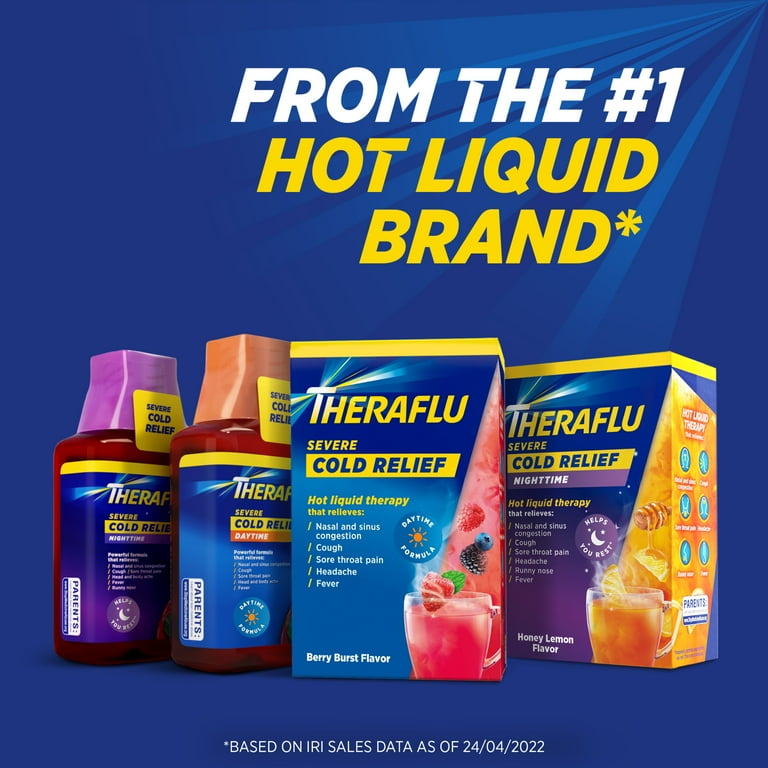This is an advertisement for Theraflu set against a blue background, featuring a white light burst from the upper right corner with streaks of paler blue emanating from it. At the top of the advertisement, in white text, it says "From the number one," followed by yellow text stating "Hot liquid brand" with an asterisk. In the center of the advertisement, there are two boxes and two bottles of Theraflu displayed.

On the left, there are two bottles: one with a purple cap labelled "Theraflu Severe Cold Relief Nighttime Formula," and another with an orange cap labelled "Theraflu Severe Cold Relief Daytime Formula." Both bottles have squared-off plastic lids and a warning for parents, although the text is unreadable.

In the center, there's a box of "Theraflu Severe Cold Relief Daytime" described as hot liquid therapy in berry burst flavor. It promises relief from nasal and sinus congestion, cough, sore throat pain, headache, and fever. The box features an image of a glass mug filled with pink liquid, adorned with a variety of berries - a strawberry, a blackberry, a raspberry, and a blueberry - falling into it.

To the right is a box of "Theraflu Severe Cold Relief Nighttime," which helps you rest and is honey lemon flavored. This box also features a glass mug with orange liquid, an orange wedge falling into it, steam rising above, and a lemon wedge behind the glass with a honey drizzle swizzle stick. There is a circle on the box with a moon icon indicating the nighttime formula.

An asterisk at the bottom of the image mentions, "Based on IRI sales data as of 24-04-2022."